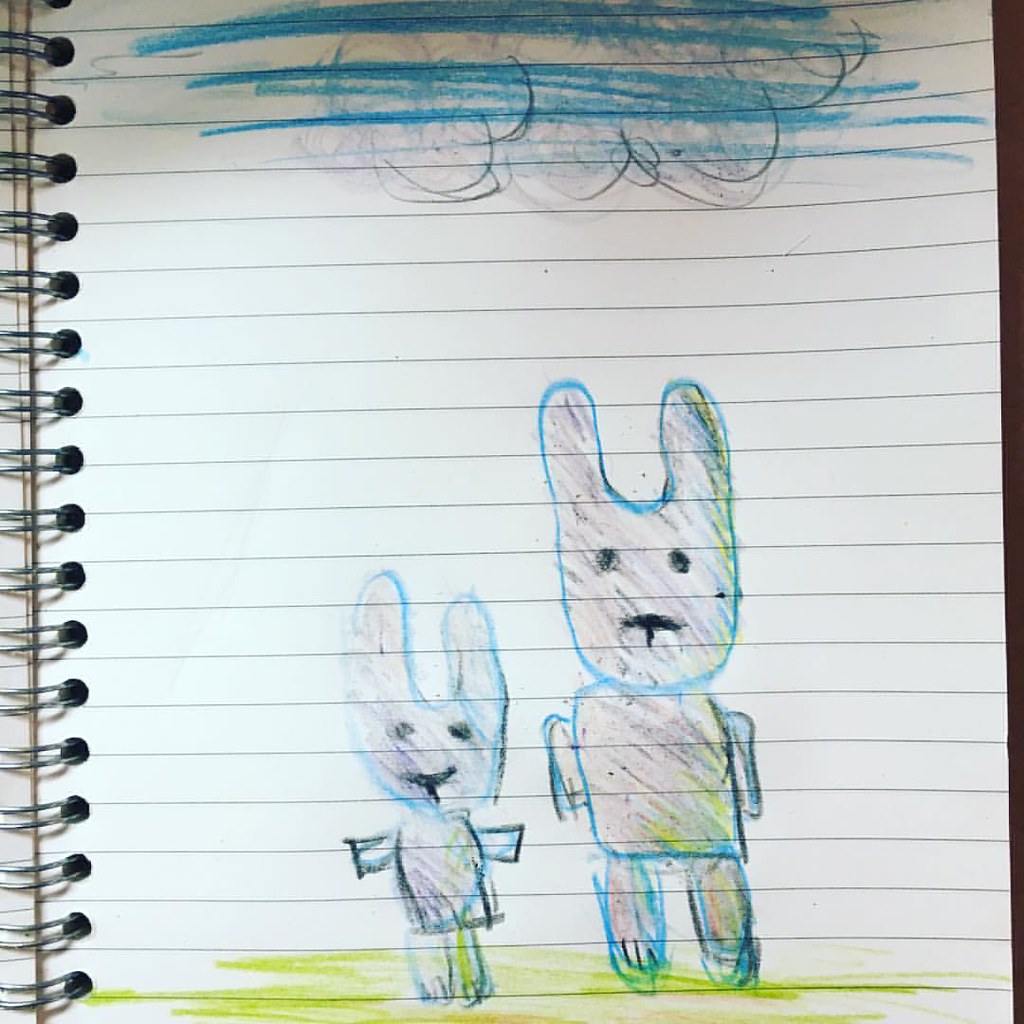This image is a color photograph of a sketch in a spiral notebook, captured in square format. The notebook features white lined paper, and the sketch is drawn on the right-hand page. The photo shows the black metal spirals running from the top left to the bottom left, holding the pages together.

The drawing, likely made with colored pencils, depicts two upright bunnies amidst a simplistic, almost child-like scene. The bunnies are predominantly brown with streaks of green and blue, and their outlines are highlighted in blue. They stand on a mustard-yellow ground which is roughly drawn. The taller bunny on the right has its arms down, while the shorter bunny on the left has its arms outstretched. Both bunnies have U-shaped heads and black circular eyes with small mouths, giving them somewhat somber expressions reminiscent of old-fashioned portraits.

Above the bunnies, there is a cloud outlined in darker lines with horizontal blue streaks running through it, suggesting a somewhat stormy sky. Additional blue lines indicate the sky behind the scene, and there are some indeterminate doodles and squiggles near the top of the page, adding to the whimsical nature of the drawing. The overall atmosphere conveys a simple, yet expressive scene that captures the viewer's interest with its unique blend of colors and shapes.